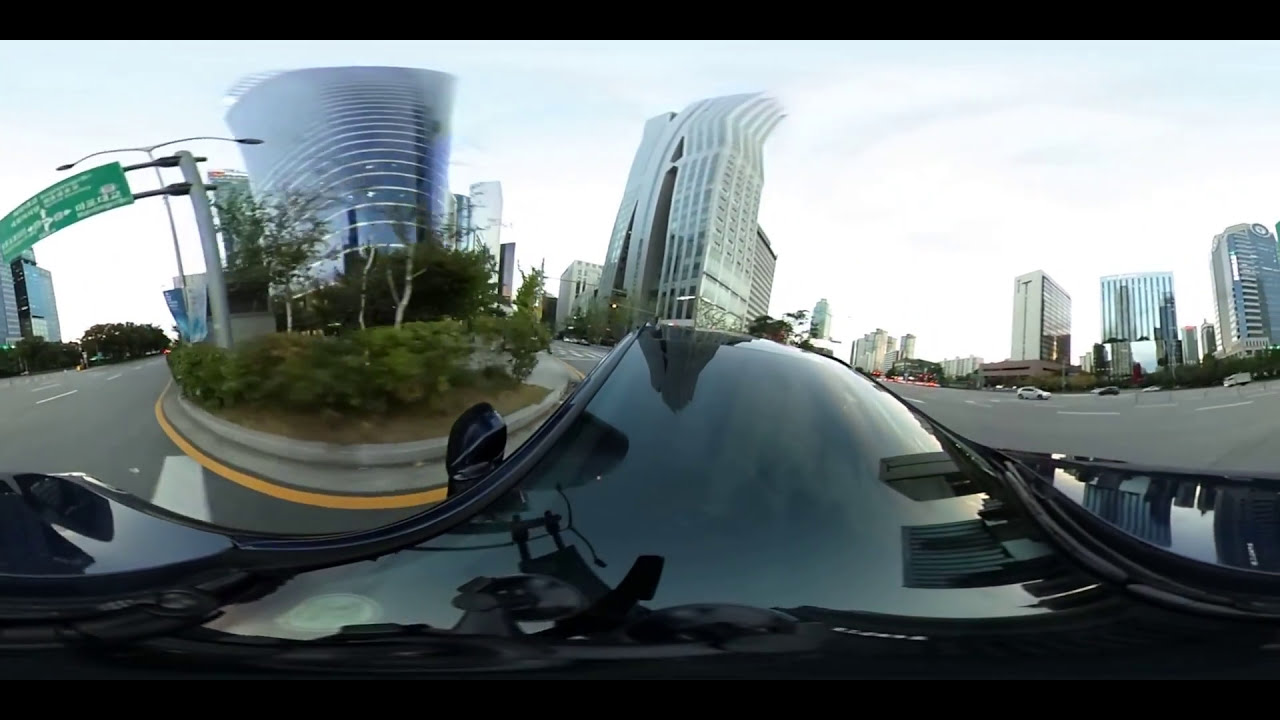The image captures an outdoor city street scene from the viewpoint of someone inside a vehicle, likely a motorcycle or car. Dominating the middle of the image are two prominent high-rise buildings, one with a bluish hue and the other white, both appearing slightly tilted due to the distorted perspective. To the right, three taller buildings and various smaller structures can be seen. The left side features green street signs, one of which might be written in Chinese, suggesting a possible location in China. The sky is overcast, casting a white, cloudy backdrop over the scene. The road visible ahead includes gray pavement with yellow and white markings, alongside a roundabout planted with small bushes and trees. Various cars, including a black one in the foreground, are driving by, adding to the busy urban atmosphere.